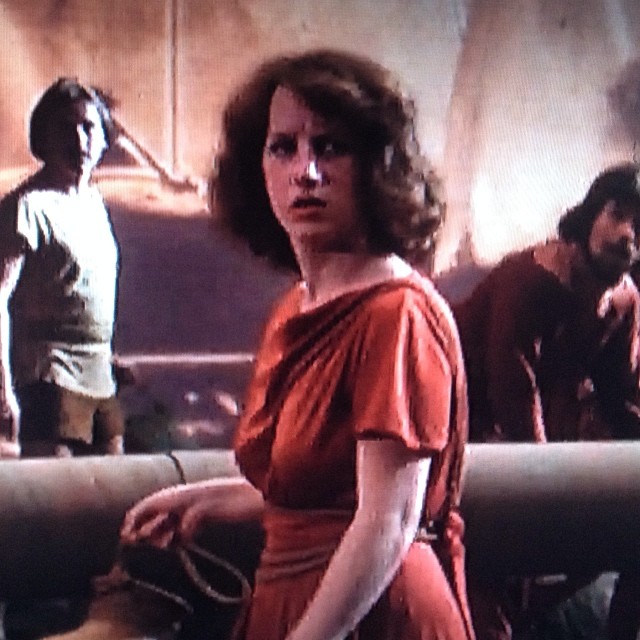The image is a blurry, grainy picture, likely taken in the 70s or 80s, featuring three individuals. At the center of the photo is a white woman with short, shoulder-length, voluminous brown hair, appearing to be in her late twenties or thirties. She is wearing a red dress and is turned to her left, looking backward with an unhappy expression. She holds a purse with its strap visible in her right hand. The background is dark, and behind her, slightly out of focus, are two men. The man on the left, also white, has dark hair and wears a light-colored shirt and brown shorts. The man on the right, also with dark hair, appears to wear a dark shirt. Both men seem to be looking in the same direction as the woman. A gray metal pipe is partially visible behind the woman on her left. The overall appearance of the image suggests that it was captured from a screen, which contributes to its distorted and low-quality nature.